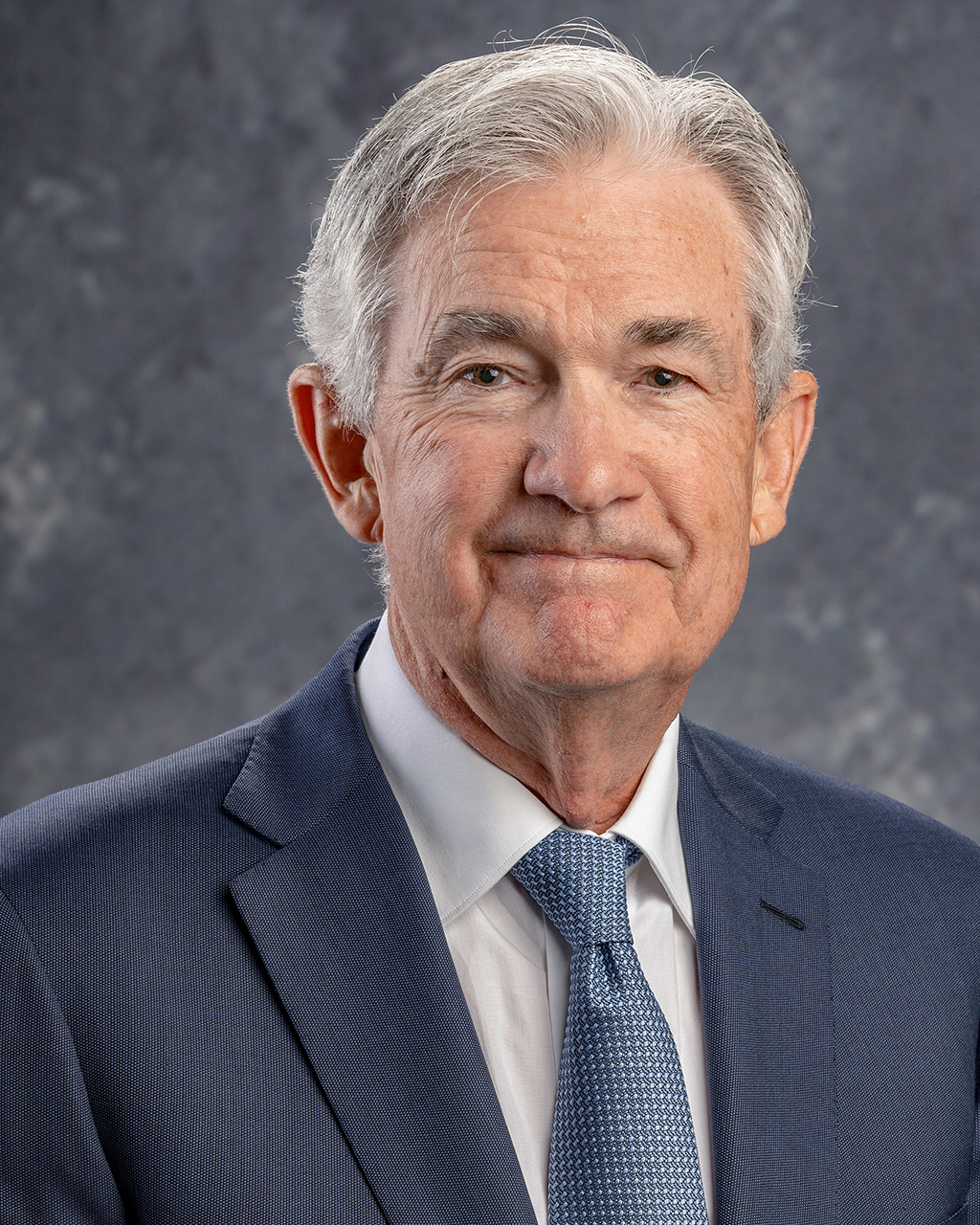This is a close-up headshot of an older man with a stately appearance. He is dressed in a dark blue suit with a white button-down shirt and a blue tie, which has speckles of white and gray. His short hair is predominantly gray, though his eyebrows retain some darker tones with hints of gray. He has hazel eyes, a clean-shaven face, and is captured with a subdued smile, without showing his teeth. The background features a gray, cloudy pattern that emphasizes his professional aura. The portrait has a bright and clear composition, making it suitable for use on a business website, magazine, or professional identification such as a lanyard.